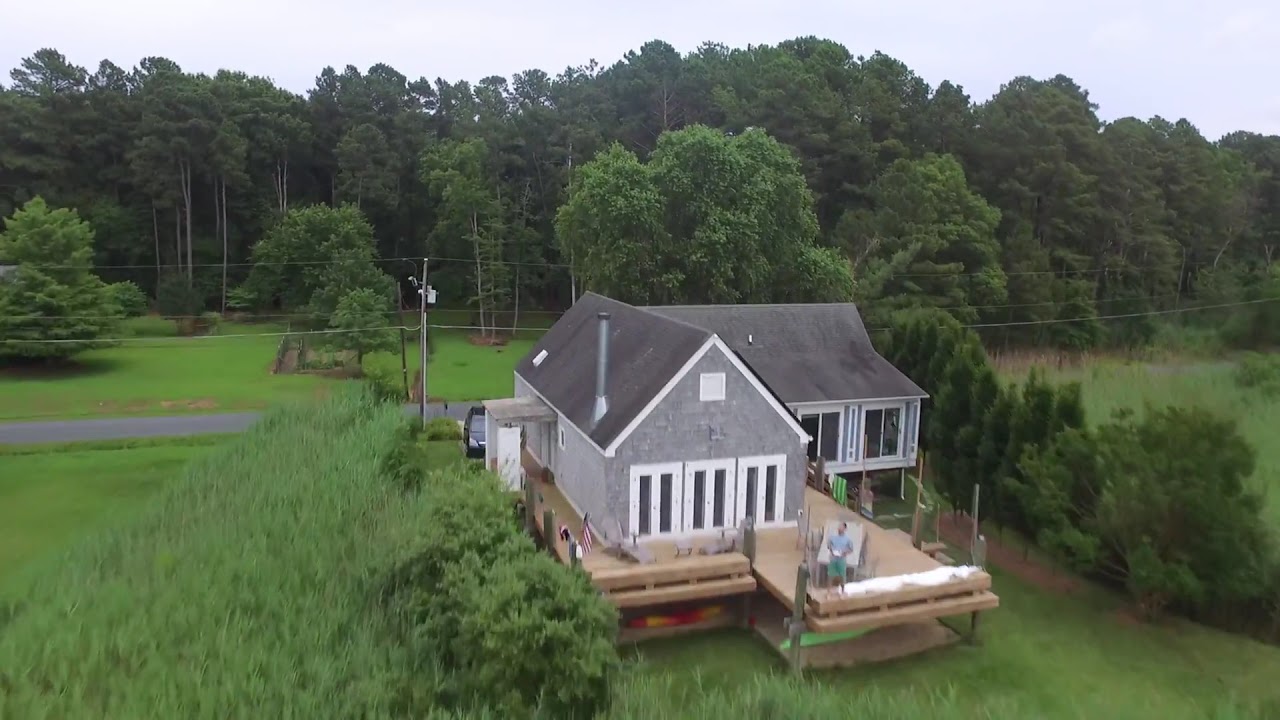The image captures a bright, sunny day where a small, elevated house is perfectly set amidst an expansive outdoor scene. The photograph shows a house that is uniquely two-toned, with the right side painted blue and the left side a light gray, both portions residing in an L-shaped structure. Elevated on a deck made of tan wooden planks, the house is supported by sturdy wooden beams. The front section of the house, facing the viewer, features a set of three windows, each with two long vertical rectangles.

A line of lush, green trees forms the backdrop, beneath a narrow strip of gray sky that suggests overcast conditions. The house is surrounded by vibrant green bushes and grass, with a narrow gray road visible on the left side, curving subtly as it leads out of frame. Centered on the front deck is a figure—small in comparison to the house—wearing green shorts and a gray-blue shirt, adding a human element to the tranquil scene. The overall composition is framed by a consistent lush greenery that enhances the secluded, peaceful vibe of this charming, wood-decked house in a picturesque setting.